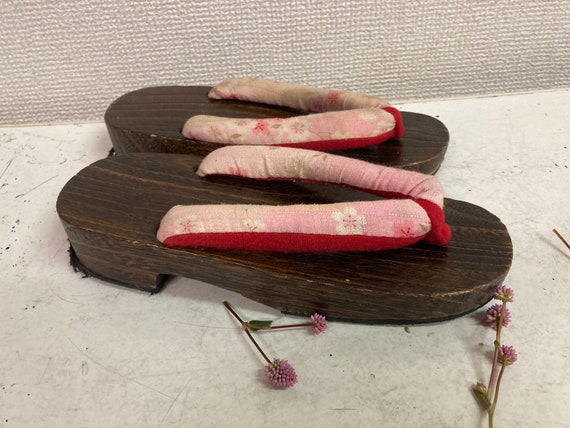The image showcases a pair of traditional Japanese geta sandals crafted entirely from solid, dark brown wood. The geta sandals feature flat tops with a carved-out heel, highlighting the distinct wooden grain and emphasizing their rigid, non-flexible nature. The soles are partially lined with felt that has started to wear away, possibly to cushion each step. The thong straps are made of puffy, cloth material with a light pink upper side adorned with a pattern of white and dark pink cherry blossom flowers, and a dark pink underside. The insoles where the toes rest are painted red. The sandals are placed on a cream-colored table that shows visible gray scratches and appears to be marble or marble-like. Accompanying the sandals, there are small pink blossoms with green stems scattered around the surface, lending a delicate contrast. Behind the table stands a wall featuring an intricate hashtag pattern, adding to the image's decorative background.